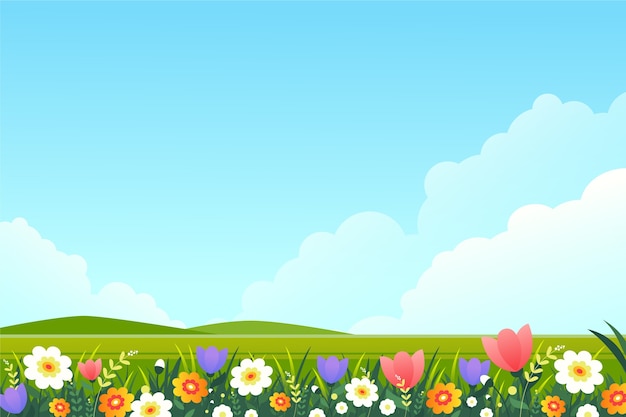The image is a cartoon-style, computer-generated scene featuring a serene landscape. The scene is predominantly composed of a light Carolina blue sky dotted with white clouds, particularly clustered near two rolling, green hills that contrast against the flat green field in the foreground. At the very forefront, a vibrant array of flowers adds splashes of color, featuring white and yellow daisies, purple and pink tulips, and other flowers in hues of orange, red, and purple. Tall grass and occasional weeds intermingle with the flowers, enhancing the natural feel of the scene. The overall simplicity and charm of the image make it ideal for use as a screensaver or background.